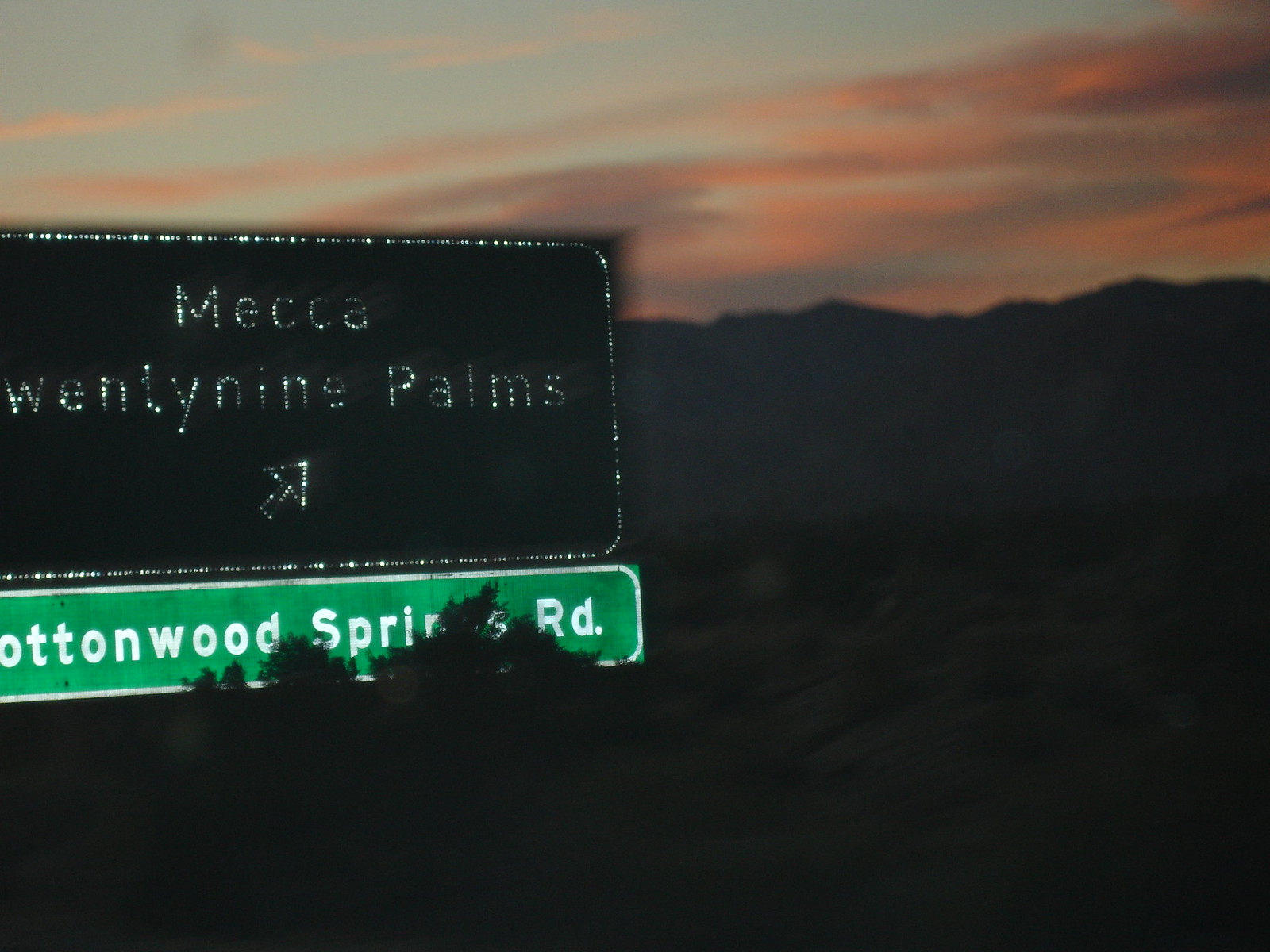This outdoor photograph captures a serene, late-afternoon scene at a crossroads. Positioned prominently on the left side are two street signs amidst some shrubbery. The lower sign is a small green, vertical rectangular one with a white border, displaying the text "Cottonwood Springs Rd" in white letters. Above it, a larger, black rectangular sign, characterized by its faded white border and lettering, partially reads "Mecca Palms," though the text on the left side is difficult to discern. A right-pointing arrow is also visible on this sign.

To the right of the signs, the landscape unfolds into dark hills, which appear nearly black in contrast to the bright sky above. The sky itself is an enchanting mix of blue and reddish hues, indicative of the sunset. Wisps of clouds add texture and further depth to the scene. The harmonious blend of the natural and man-made elements makes for a captivating and tranquil image.